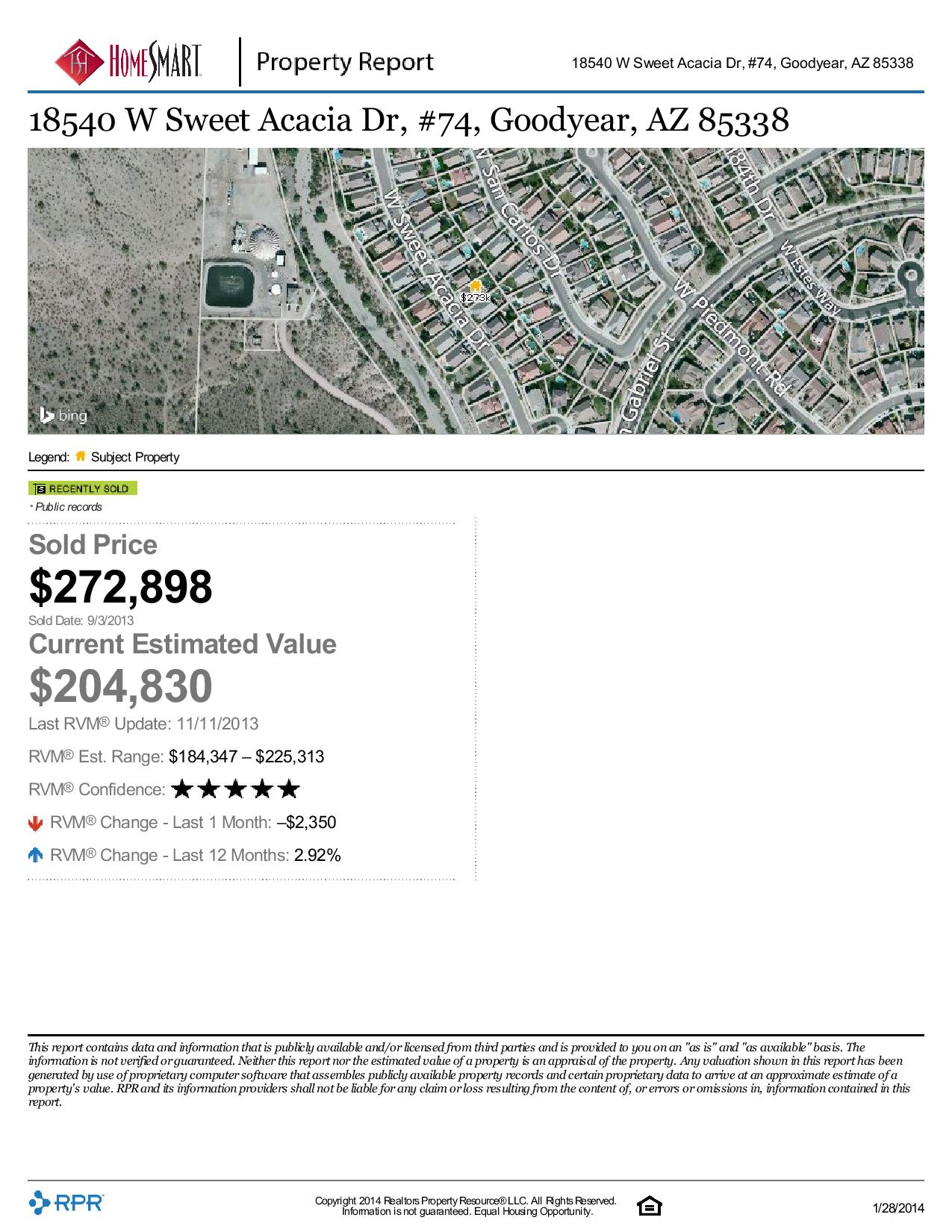**Detailed Home Listing Image Caption:**

This home listing image features a white background with black text and an overhead satellite photograph of a neighborhood. 

In the upper left-hand corner, there's a red diamond logo with an outline drawing of a house, labeled "HomeSmart." The word "Home" is in red, while "Smart" and the following text "Property Report" are in black. 

On the upper right-hand side, the text reads "18540 West Suite Acacia Drive, Unit #74, Goodyear, Arizona 86338" in black, and it's followed by a blue horizontal line. 

Below the line, the address "18540 West Suite Acacia Drive, Unit #74, Goodyear, Arizona 86338" is repeated in larger black text. 

Beneath the address, there is an overhead satellite photograph sourced from Bing, as indicated by the Bing logo and the word "Bing" in the lower left-hand corner of the image. The photograph depicts a suburban neighborhood with clearly labeled houses and streets.

Below the satellite image are the detailed metrics of the home listing:
- **Home Sold Price**: $272,898
- **Current Estimated Value**: $204,830
- **Last RVM Update**: November 11, 2013
- **Estimated Range**: $184,347 to $225,313
- **Confidence Score**: Five stars

This comprehensive listing provides essential information including past sale price, current value estimates, and the confidence in the evaluation.